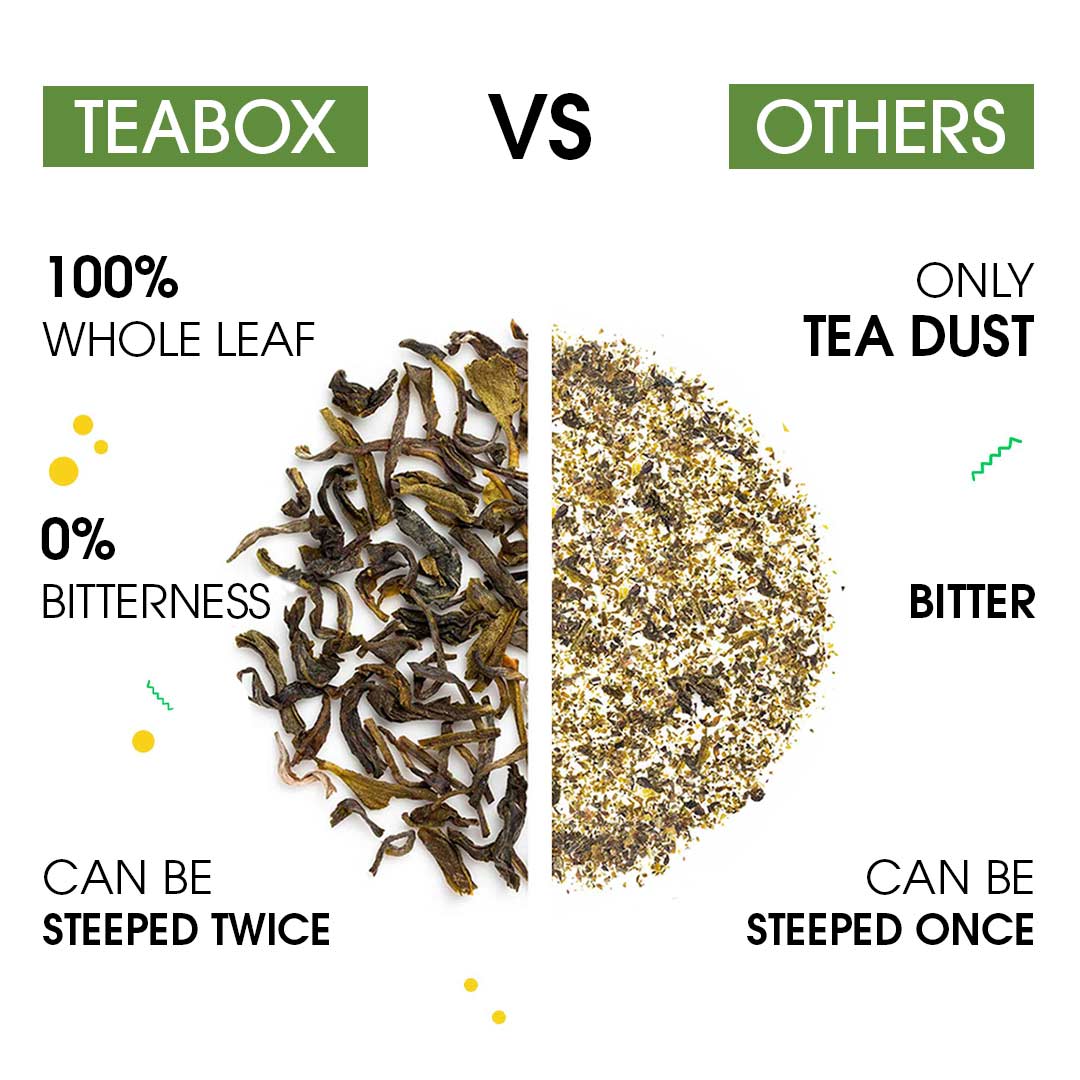This minimalist infographic, set against a completely white background, contrasts the quality of tea featured in a "T BOX" with others. At the very top, bold white letters in green rectangles label the sections: "T BOX" on the left and "OTHERS" on the right, separated by a black "VS" in the center. In the middle of the image is a circular visual, split down the middle. The left half displays 100% whole, dark brown tea leaves, while the right half shows finely powdered tea dust of a similar brownish hue. Below "T BOX," it states, "100% Whole Leaf, 0% Bitterness, Can Be Steeped Twice," accentuated by small design elements such as circles and a yellow circular motif with green squiggles. On the "OTHERS" side, it reads, "Only Tea Dust, Bitter, Can Be Steeped Once," with a small green squiggly line among its minimalistic elements. The overall comparison highlights the superior quality of whole leaf tea in the T BOX as opposed to the inferior tea dust found in typical tea products.